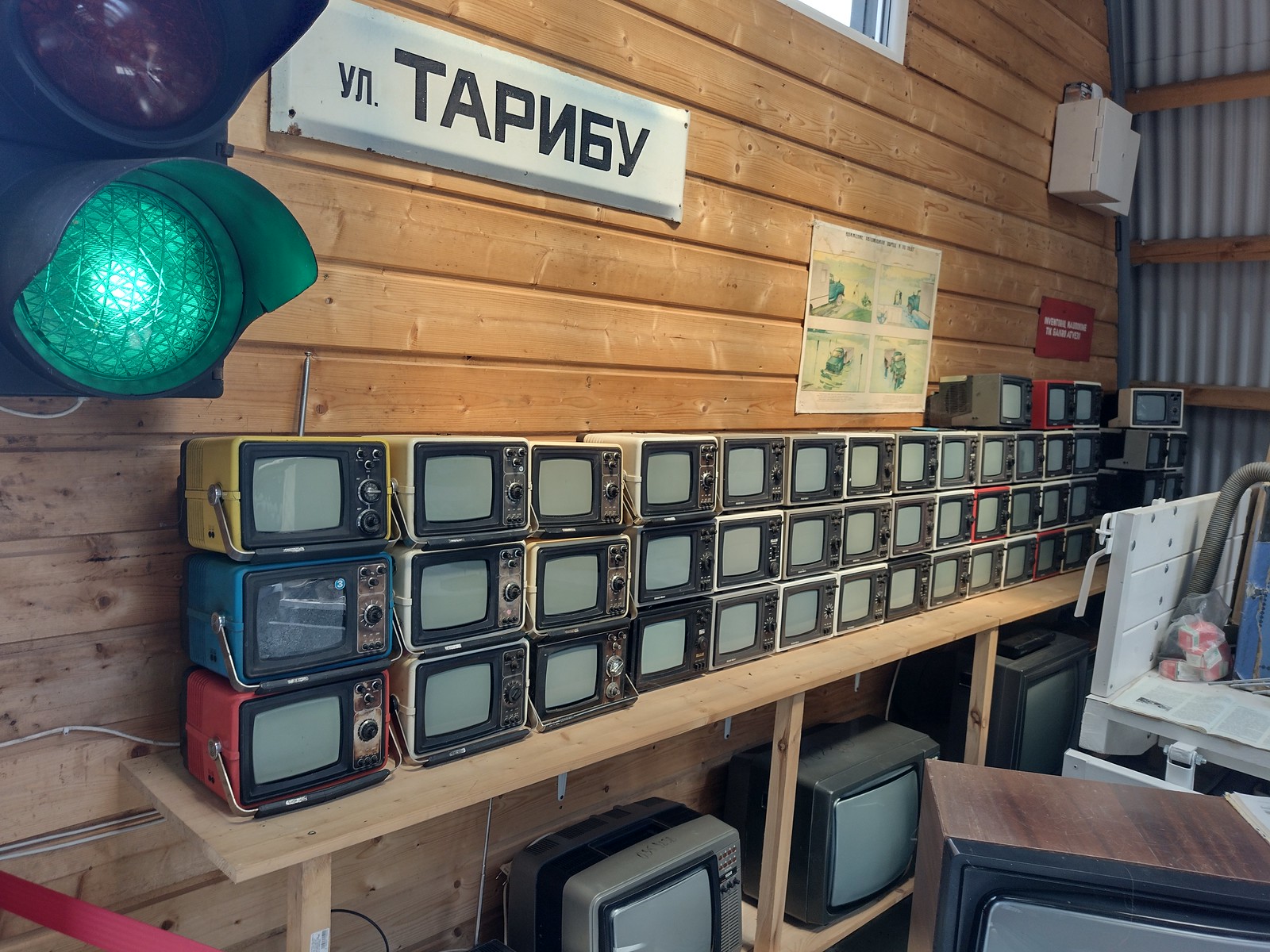The color photograph depicts a captivating assortment of vintage tube-style televisions arranged meticulously on a wooden shelf. The shelf, set against a light brown wooden backdrop, holds a variety of portable televisions with brightly colored casings in yellow, blue, and red, all featuring gray screens. Below these small TVs, the lower section of the shelving unit displays medium-sized, antique-looking gray and black televisions with prominent backs.

On the upper left corner of the wall, a green-lit traffic light hangs, accompanied by a white sign with ambiguous black lettering, which appears to be in Russian. The background of the sign is white, presenting a mix of familiar and backward letters resembling "TAP" and "6y". Adjacent to this, a white poster with indistinct greenish images and a few other signs and boxes are scattered across the wall, adding to the eclectic visual appeal. The right-hand corner features an iron or aluminum sheeting intersected by wooden or aluminum beams, contributing a unique texture beneath more traditional wooden panelling. The detailed display conveys a nostalgic charm through its array of colorful, old-fashioned tube televisions, contrasting signage, and the curious assembly of various wall elements.